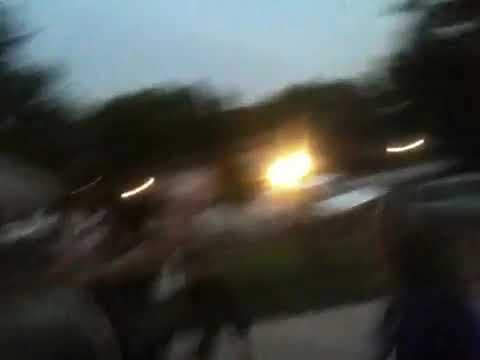The image is extremely blurry, making it difficult to discern specific details. It appears to have been taken outside during the evening. The sky at the top displays a light blue color, transitioning to darker shades as the evening progresses. Illuminated by a bright light source, likely a street lamp, the scene reveals vague silhouettes, possibly of trees, people, and cars. The bright yellow spot in the center of the image suggests an artificial light, casting a whitish burst against the blurred background. The entire image is a blend of beige, gray, green, blue, and black hues, with the colors smearing across the picture as if it was captured in motion. The bottom of the image shows a light-colored area, possibly part of the street, accompanied by hints of green. Despite the blur, it’s evident that objects and individuals populate the scene, with people presumably on the left side and cars in the middle.